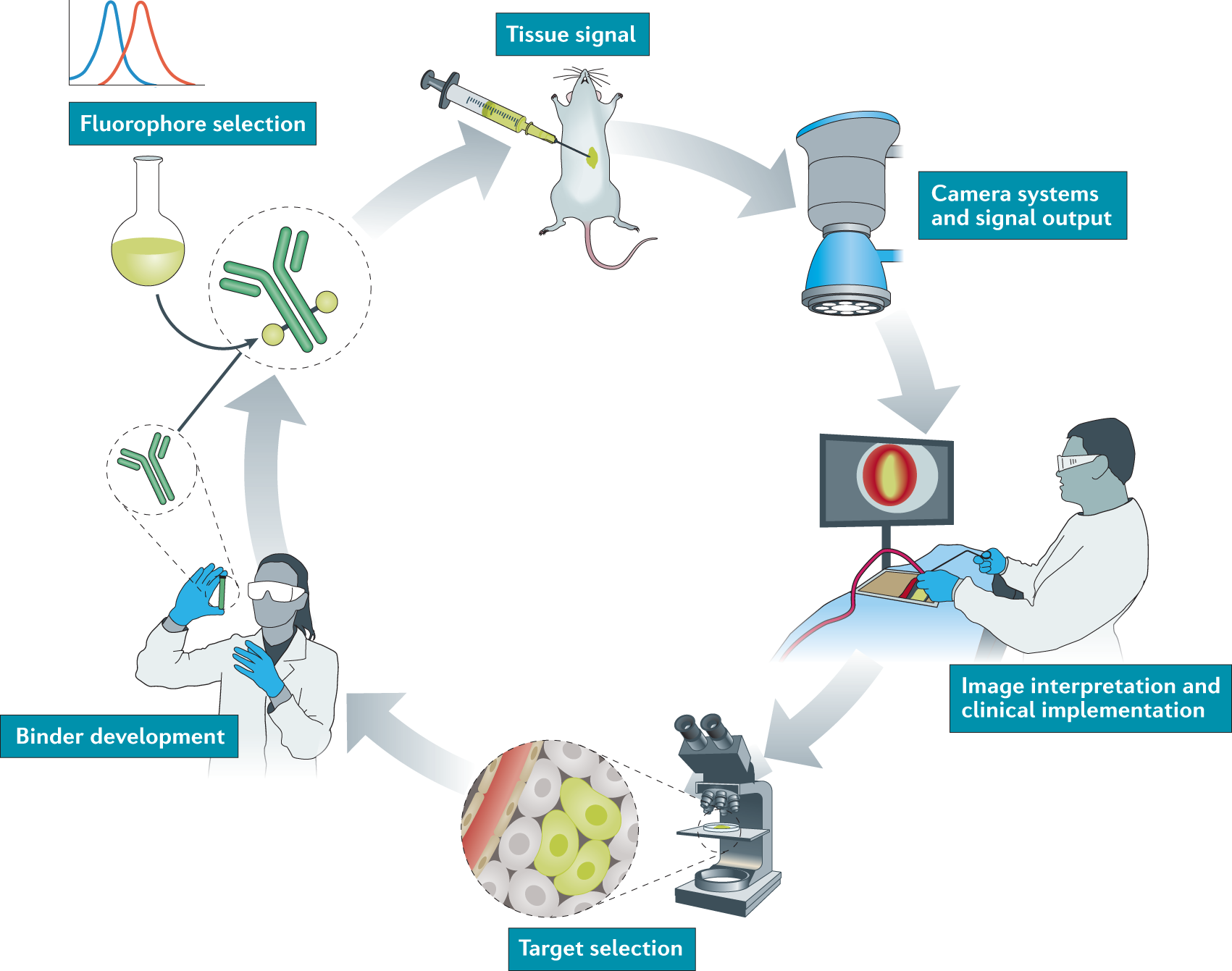The image is an infographic designed in a circular format with arrows creating a continuous loop, all pointing clockwise. The arrows are curved and colored gray, forming the outer structure of the circle. Positioned within each arrow is a light blue rectangle containing white text and an icon, illustrating different stages or components of the process.

At the top, the first section is labeled "Tissue Signal." This part features a needle injecting yellow or green liquid into the belly of a mouse that is lying on its back. Moving clockwise, the next section is titled "Camera Systems and Signal Output," depicted with a light blue and gray camera. Further down, the section "Image Interpretation and Clinical Inflammation" is highlighted, showing a man wearing glasses and seated at a desk with a computer screen. The screen is gray with a red and yellow symbol at its center.

Additionally, another section labeled "Fluorophore Selection" involves a depiction related to germ analysis. Each label and icon serves to represent a distinct stage in the process, presented in clear blue-green rectangles with white text. Together, these detailed icons and descriptions illustrate a scientific cycle, potentially related to medical or research fields, emphasizing the interconnected steps from tissue signal acquisition to image interpretation and germ analysis.